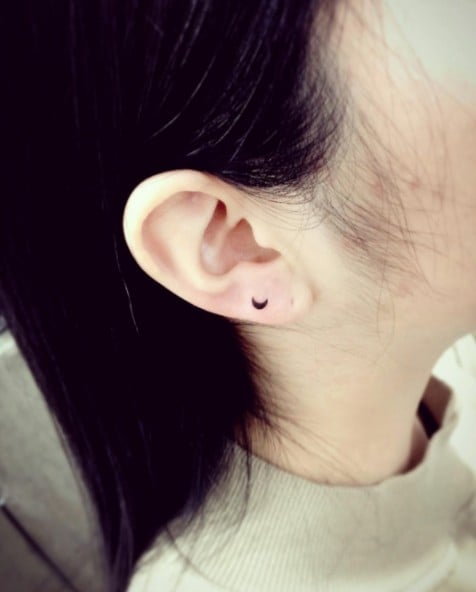This image depicts a close-up of the right side of a woman's head and neck. The woman's complexion is light, and her straight, dark hair—either black or dark brown—is neatly tucked behind her ear. Her profile reveals just the side of her face, ear, and neck, with her face obscured from view. She is wearing a beige, almost turtleneck-like sweater with a collar that fits snugly but not too tightly against her neck.

Her ear features two piercings: the lower earlobe has an empty hole, and the upper lobe sports a distinctive black crescent moon-shaped earring. This earring appears almost like a tattoo but is indeed an earring. The background of the image is unclear but suggests she might be leaning against a gray object, which could be a pillow, cushion, or the backrest of a chair. The overall scene captures a serene and detailed focus on the accessories and textures, highlighting the simplicity and elegance of her appearance.